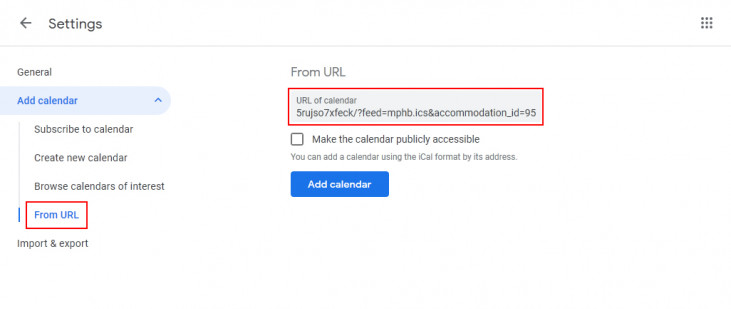This screenshot showcases the settings page of an unidentified calendar application. At the top is a header bar with the word "Settings" prominently displayed. Adjacent to this, there is a back button and a box icon with three dots indicating more options. Below the header, a thin gray line separates the top section from the main content.

The left side of the screen begins with "General" in black text. Below this is "Add Calendar" highlighted in blue with a light blue bubble around it. Under this section, there are options listed in sequence: "Subscribe to Calendar," followed by "Create new calendar," and "Browse calendars of interest."

Further down, a red-lined box contains the option labeled "From your URL," with "Import and Export" written in black text beneath it. On the right side, the phrase "From URL" appears in gray text. Inside another red-lined box with a gray interior, there is a field labeled "URL of the calendar" where the calendar URL can be entered. 

A checkbox below this field allows the user to make the calendar publicly accessible, indicated by gray text. A small note below this checkbox reads, "You can add a calendar using the iCal format by its address."

Finally, at the bottom, there is a blue bar with white text that reads "Add Calendar," which can be clicked to finalize the addition of the calendar.

The page primarily uses a white background with accents of red and blue to highlight interactive elements.